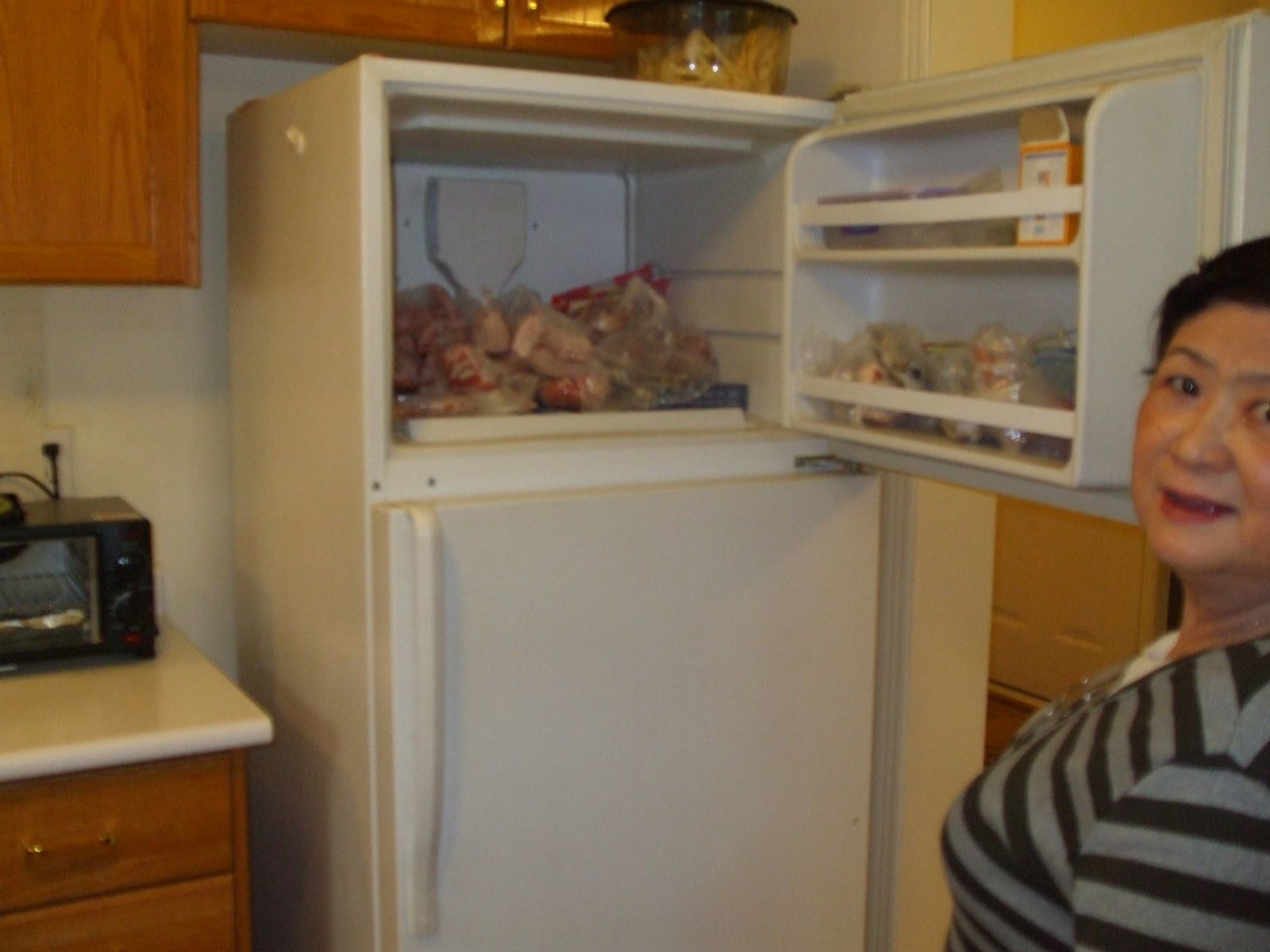In the kitchen, an Asian woman with short, dark hair stands in front of an older white refrigerator, the top freezer door open to reveal an array of clear bags containing frozen foods, possibly meats, and an orange box. She is dressed in a black and gray striped shirt and is looking over her left shoulder while smiling at the camera. The kitchen features medium brown cabinets above and below the refrigerator, a white countertop, and a black toaster oven plugged in and situated on the counter to the left. The image portrays a cozy, somewhat dimly lit kitchen with a gently worn, homely atmosphere.